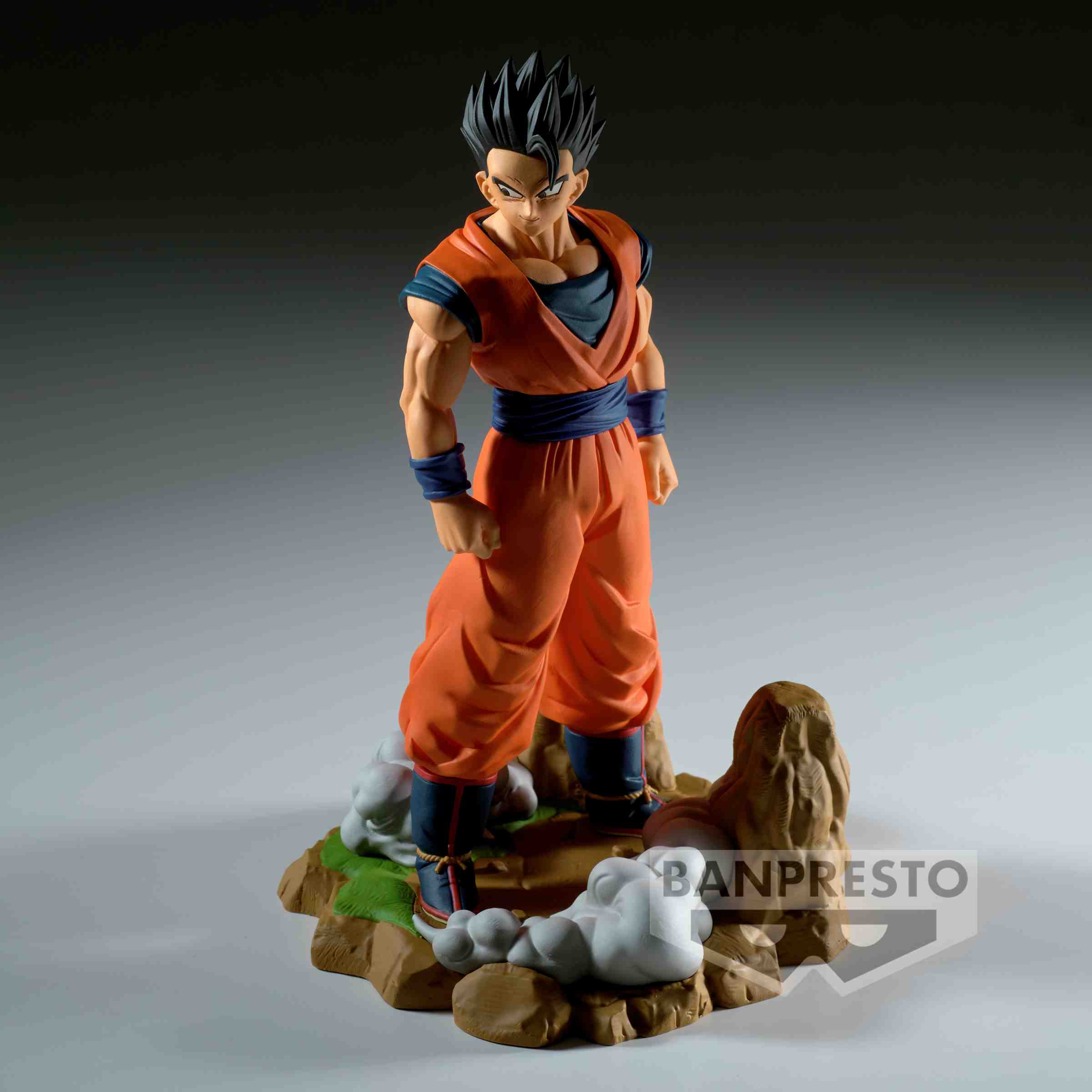The image depicts a highly detailed and muscular figurine of Adult Gohan from the Buu Saga of Dragon Ball Z, produced by Banpresto. The figurine, designed for display rather than play, stands prominently on a textured base resembling a small island or rocky outcrop. Gohan is posed confidently, with his chest facing the right and head looking straight ahead, exuding a fierce and determined expression. He sports his classic orange and dark blue gi, spiky black hair, and lean physique. The backdrop features a gradient effect transitioning from black at the top to light gray at the bottom, complemented by the superimposed Banpresto brand name and a stylized, rotated bee symbol. There are no other characters or additional elements in the background, ensuring that Gohan remains the focal point of this striking collectible.